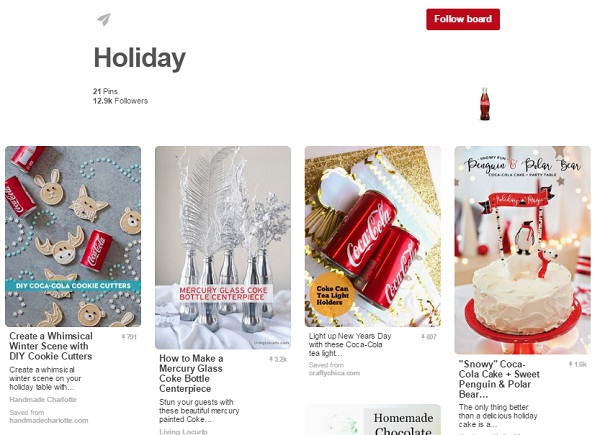The image depicts a Pinterest holiday board featuring 21 pins and boasting 12.9K followers. In the top right corner, there's a prominent red "Follow Board" button. Adjacent to it, a small Coca-Cola can icon is visible. The central area of the image showcases four vertically oriented, large rectangular pin ideas, predominantly themed around Coca-Cola.

On the far left, there's a pin for DIY Coca-Cola cookie cutters, featuring Coca-Cola cans and cookies, with the text "Create a whimsical winter scene with DIY cookie cutters." 

Next to it is a pin explaining how to create mercury glass Coke bottle centerpieces, displaying silver bottles adorned with flowers and greenery.

To the right of that, another pin shows Coca-Cola tea light holders, with the caption "Light up New Year's Day with these Coca-Cola tea light holders."

On the far right, a pin features a snowy Coca-Cola cake topped with a penguin and polar bear, described as a "sweet penguin and polar bear."

Each pin captures a festive, Coca-Cola-inspired creative idea, perfect for holiday celebrations.